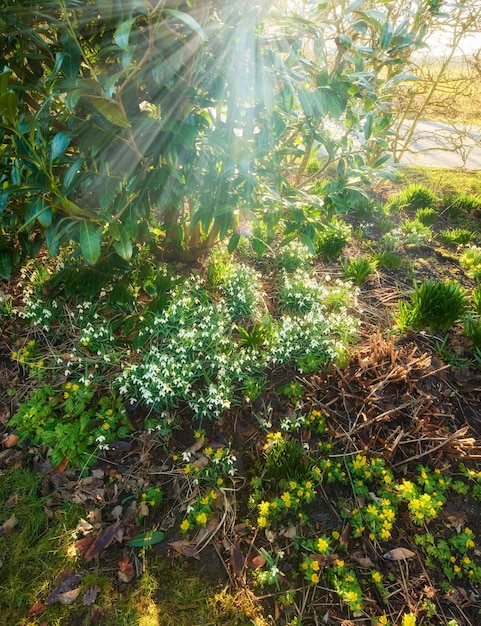A photograph taken from standing height features a lush, vibrant scene where a variety of plants and flowers flourish along a narrow, asphalt-covered pathway. The top left corner is dominated by a larger bush with long, oval-shaped green leaves that hang downward, casting speckled shadows on the scene below. Light beams from the sun shine from the top center of the image, creating a golden glow that illuminates the landscape. The bottom two-thirds of the photograph focuses on the ground, revealing dark brown dirt interspersed with dried grasses, clumps of green grass, and clusters of small yellow and white flowers. The white flowers, resembling delicate insects with white wings, and the vibrant yellow flowers are clearly segregated into their own distinct groups, adding splashes of color to the earthy tones. On the right side of the image, a grassy border extends towards what appears to be a shimmering body of water, enhancing the photo's serene and picturesque atmosphere.